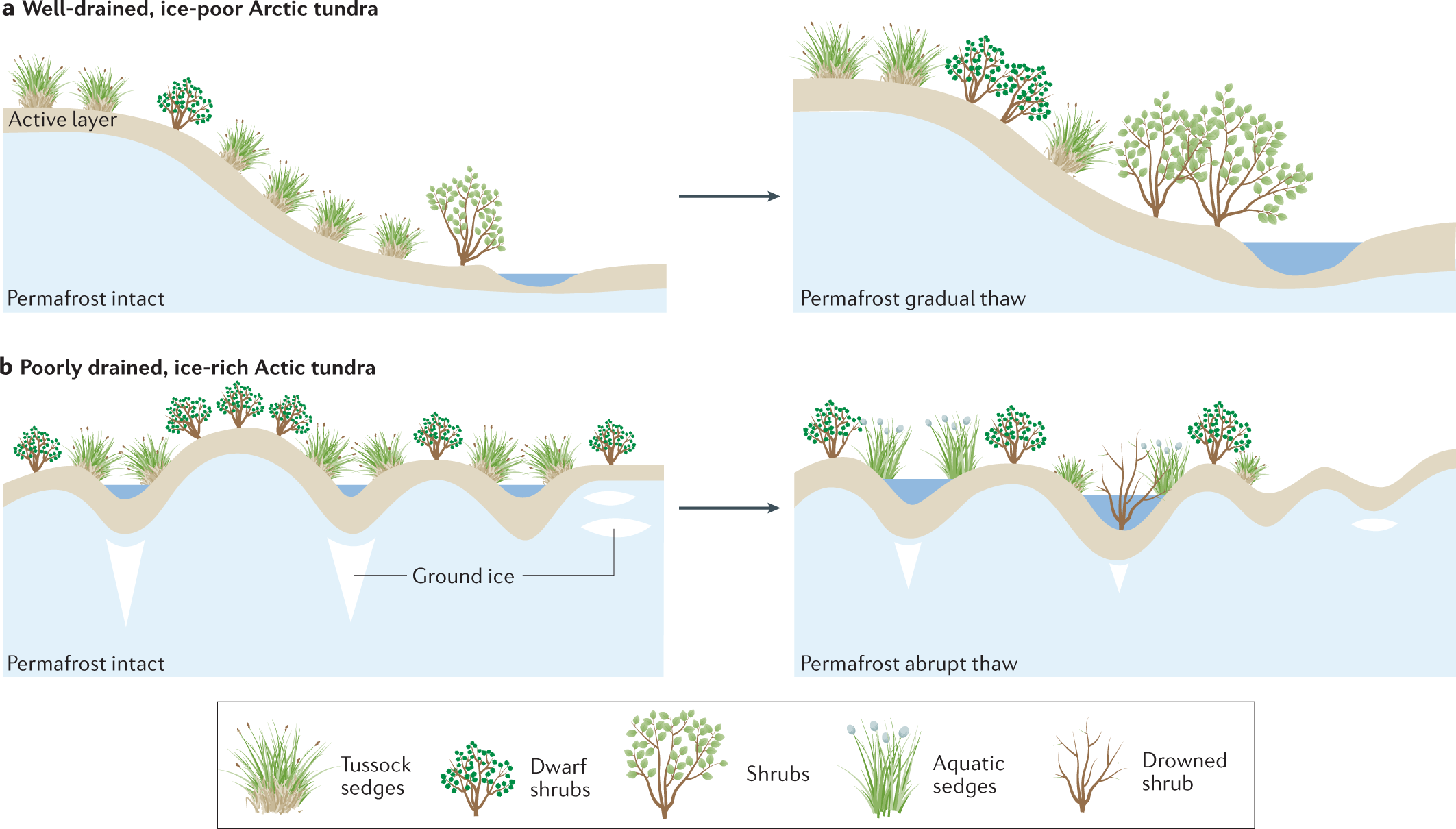This is a detailed digital information image that illustrates various stages of Arctic tundra conditions and plant life. The image is set against a white background and contains four main drawings organized in two rows and two columns at the top, with explanatory text and illustrations of plants at the bottom.

In the top left drawing, labeled "Well-Drained Ice-Poor Arctic Tundra," we see a surface area with green-leaved plants growing on a brown active layer. Below this active layer is a blue section marked as "Permafrost Intact." An arrow points to the right from this drawing to the next.

The top right drawing, similar to the first, shows the active layer getting thicker and is labeled "Permafrost Gradual Thaw." 

The bottom left drawing depicts a more complex scene with a highly curved active layer and white spots within the blue permafrost layer labeled "Ground Ice." 

In the bottom right drawing, the white spots within the blue permafrost layer vary in shape and number and it is labeled "Permafrost Abrupt Thaw." 

At the bottom of the image, there are additional drawings of various plants such as tussock sedges, dwarf shrubs, aquatic sedges, and drowned shrubs with their names clearly written.

This comprehensive and visually structured image effectively communicates the stages and types of Arctic tundra and plant developments through a combination of detailed drawings and descriptive text.